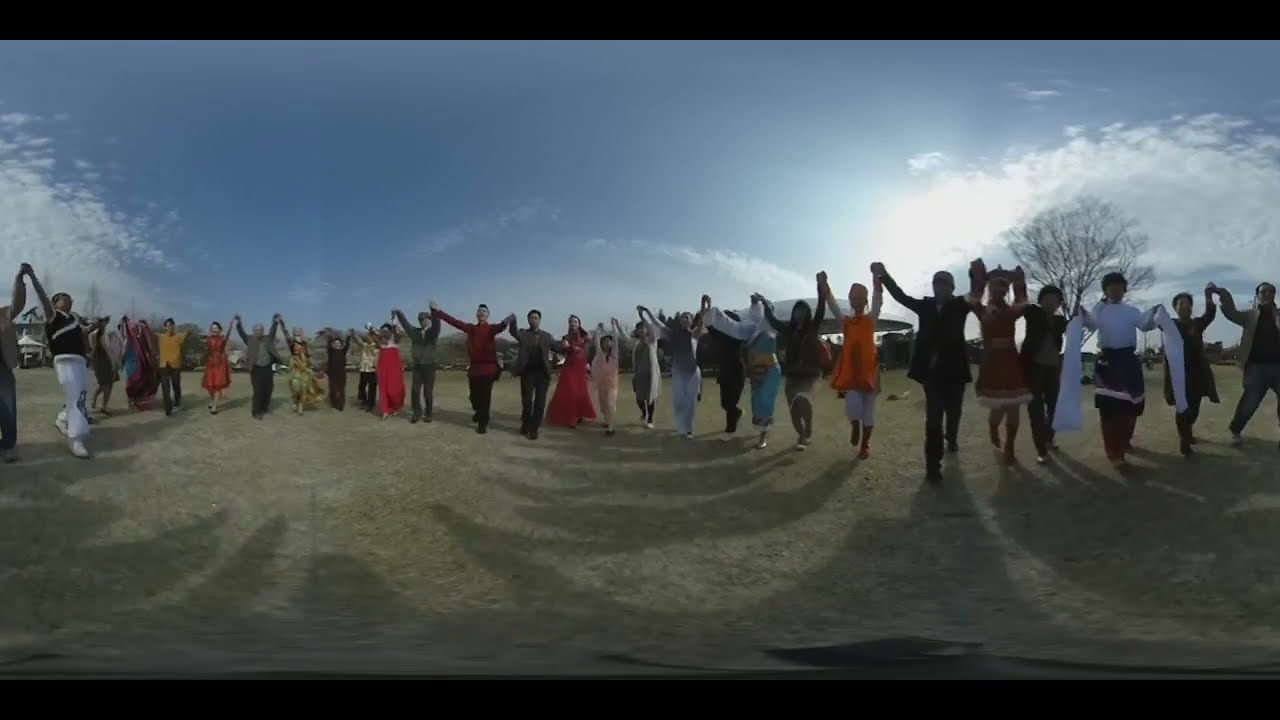In this detailed outdoor scene, a long line of roughly 30 people stands hand-in-hand, stretching across the center of a wide, open field with short grass. This celebratory gathering features men, women, and perhaps a few children, all facing the camera. Most appear to be Caucasian and are dressed in traditional clothing, suggesting an ethnic celebration. Among the garments, some women wear white blouses with blue skirts, others don red traditional dresses, and some men are dressed in more formal attire, including business suits. The image is captured in the middle of the day under a bright blue sky with few scattered clouds, though the sun is slightly obscured, casting shadows across the scene. The backdrop includes some distant outbuildings and perhaps parked cars, indicating a rural or semi-rural setting. The people, joyous and celebratory, hold their hands up, creating a sense of unity and festivity amid the vibrant mix of black, blue, gray, white, red, yellow, orange, tan, and light blue hues around them. The image has a black border framing the lively scene.